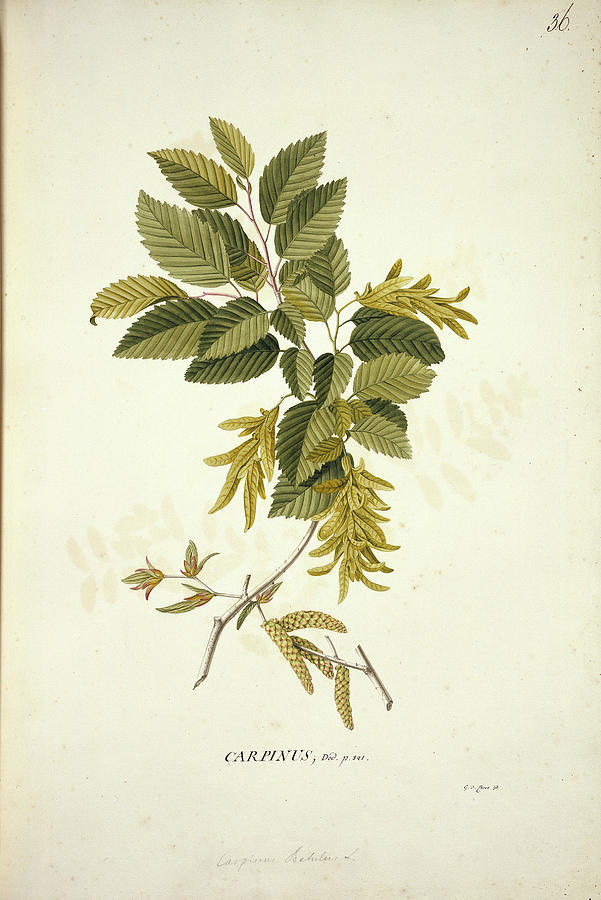This detailed colored illustration depicts a single sprig of the plant Carpinus against a yellowish background. The main stem, which is gray and subtly curved, runs through the center of the image and extends towards the right before bending back to the left. Multiple smaller branches emanate from the stem, each sporting ovate leaves that taper to a pointed tip. The leaves are richly textured with prominent V-shaped veins and have serrated edges. They come in two primary colorations: a mix of darker and lighter green halves, as well as uniformly light green leaves. Some of the leaves appear yellowish and withered, suggesting stages of decay. Additionally, there are branches with clusters of cone-like projections near the base, reminiscent of budding seeds poised to propagate new plants. A tiny flower is also visible on a minuscule branch to the left side of the main stem. Below the plant, the text labels it as Carpinus. The background subtly highlights the plant's features, with shadows cast from the leaves reinforcing their three-dimensional form. The entire illustration resembles an excerpt from a detailed botanical or science book, with accompanying, although unreadable, textual facts.